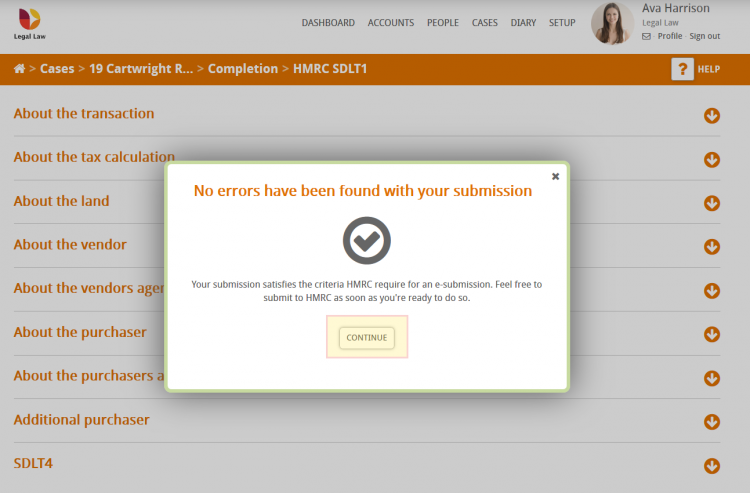**Detailed Caption:**

The image depicts Ava Harrison logged into the Legal Law platform. The website's interface prominently displays a navigation bar across the top with tabs labeled: Dashboard, Accounts, People, Cases, Diary, and Setup. Currently, Ava's profile is highlighted, possibly indicating she is managing her account or settings. The main workspace is divided into sections, with the left side showing shortcuts for 'Home' and 'Cases.'

One active case, titled "19 Cartwright Completion," is selected, revealing its unique code. A prominent display screen in the background informs Ava that her submission has been successfully reviewed, stating, "No errors have been found with your submission. Your submission satisfies the criteria HMRC requires for an e-submission. Feel free to submit to HMRC as soon as you're ready to do so." Below this message, there is a 'Continue' button, guiding users to proceed with the next steps.

In the background, several dropdown menus provide further details that need to be addressed, including information on the transaction, tax collection, land details, vendor details, vendor’s age, purchaser details, an item that begins with an 'A,' and additional purchaser information. These dropdowns allow for further customization and input as necessary. While the current state of the interface suggests that Ava may need to complete other sections before submission, the platform appears user-friendly, enabling easy navigation and edits as needed.